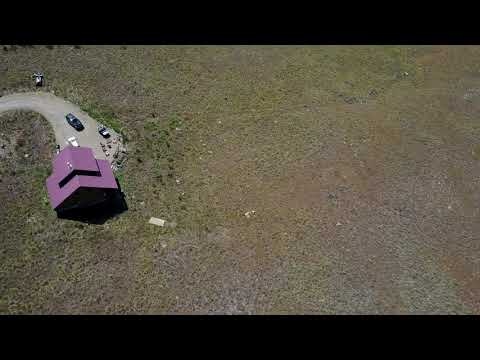This aerial photograph, captured from a height of approximately 100-300 feet, showcases an isolated hillside dominated by a large field of grass interspersed with patches of brown and green, suggesting a mix of vegetation and possibly some rocky terrain. Central to the image, positioned on the left side, is a lone house or possibly a large barn with a distinctly large purple roof. This structure appears modest in size, akin to a rancher with a slanted roof. In the driveway in front of the house, three cars are parked, hinting at some human activity, though no people are visible. The remaining landscape is predominantly green with some areas not as lush, reflecting the natural wear and seasonal shifts of the terrain. The top and bottom edges of the image are marked by darker brown bands, and the overall setting suggests a sunny day. The scene conveys a sense of solitude, with minimal human structures amidst the expansive grassy hillside.